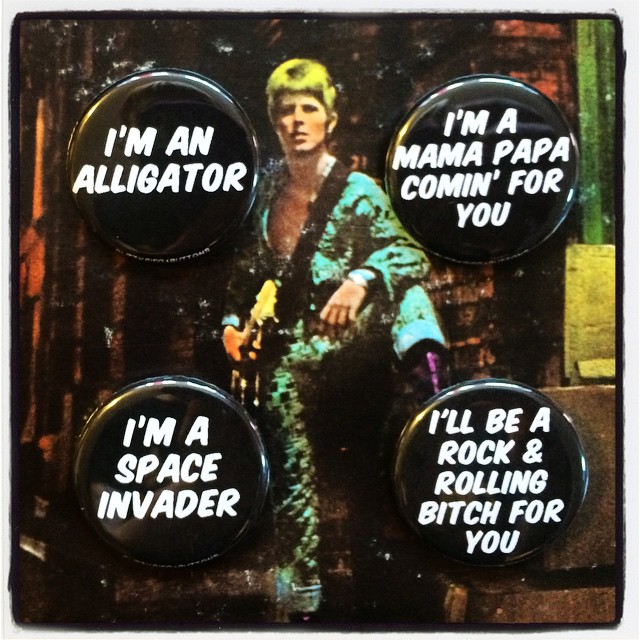This image showcases an artistic mix of painting and mixed media elements centered around a vintage, grainy photograph of a Caucasian musician with blonde hair, standing on stage with one leg up on a speaker. The musician, depicted in a striking green jumpsuit with the shirt unbuttoned to reveal his chest, and donning purple boots, holds a guitar strapped over his shoulder. He stands confidently in front of a brick building with some industrial designs visible in the background. The entire scene is framed within what appears to be a coaster.

Overlaying this vintage visual are four glossy black buttons with white text, placed in each quadrant of the image. The top-left button reads, "I'm an alligator"; the top-right says, "I'm a mama papa coming for you"; the bottom-left reads, "I'm a space invader"; and the bottom-right states, "I'll be a rock and rolling bitch for you," possibly referencing the musician's song lyrics. The contrast between the aged photograph and the glossy buttons creates an intriguing, layered composition.